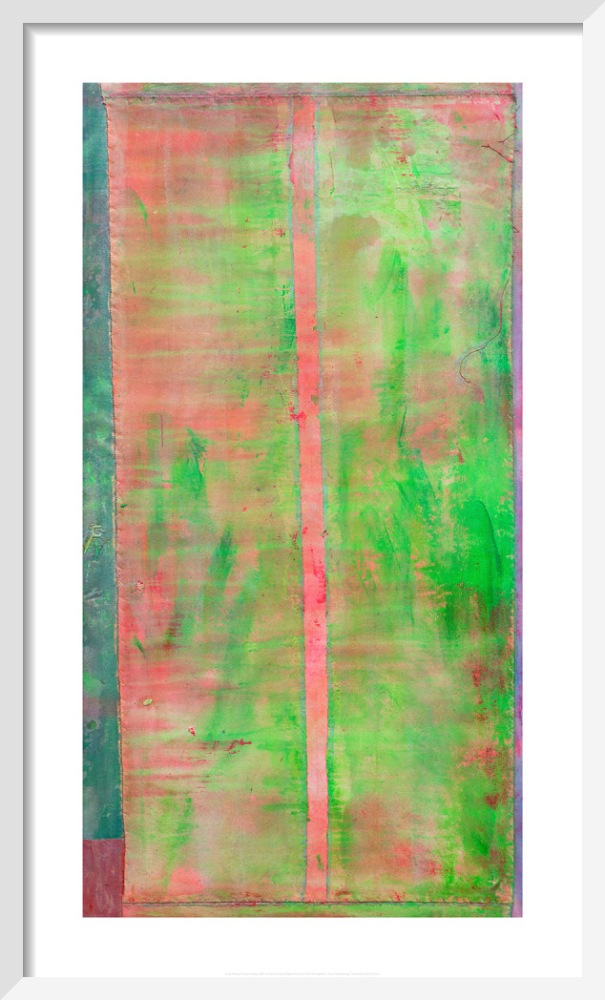The image depicts a tall and narrow abstract painting characterized by its vibrant and dynamic color scheme. Dominated by neon green and bright red hues, with a prominent, thick vertical stripe of neon pink cutting through the center from top to bottom, the painting offers a striking visual contrast. The right side predominantly features bright green and red tones, whereas the left side transitions into darker shades, including a maroon and a bluish color. Additional elements include streaks and splotches of neon green, a vertical strip of teal on the left edge, and a dark red square at the bottom left corner. The background appears digitally added, framed with a sleek, light gray border and white surrounding, hinting at a digitally generated frame. Patterns within the painting are varied and abstract, adding to the depth and complexity of the composition.